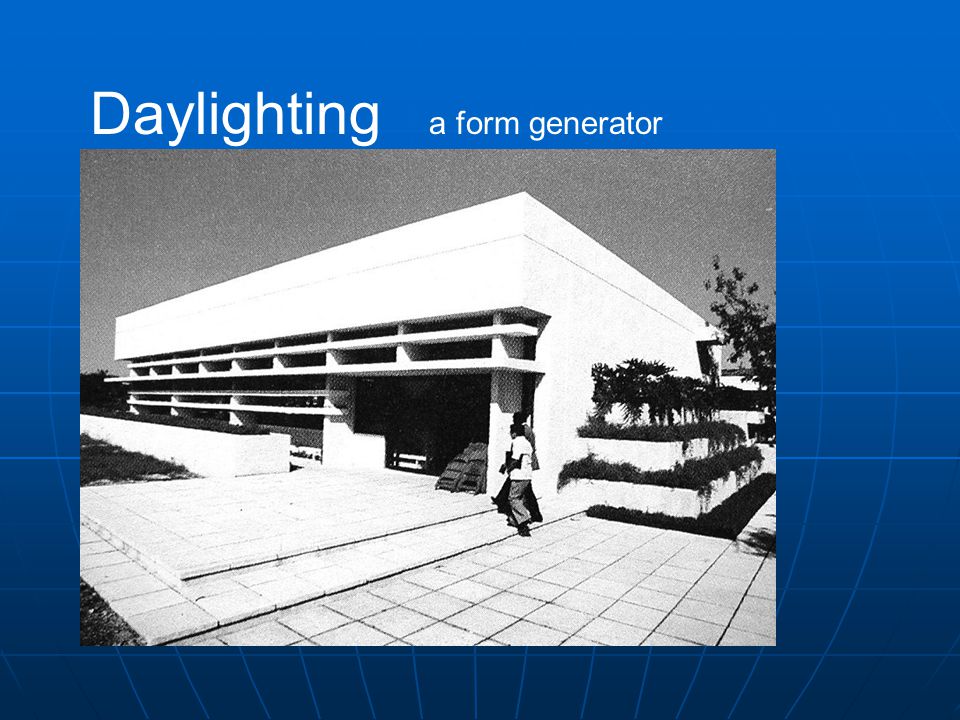A black and white photograph features a modern, one-story white office building with a unique architectural design. The image, set against a deep blue-black background, is outlined with a blue frame and titled at the top in large font: "Daylighting, a Form Generator." The building facade is characterized by cutout sections and open rectangular spaces that resemble window openings devoid of glass. The front entrance, marked by a black door, is approached by two men ascending two steps. The entrance area, somewhat like an outdoor foyer, shows a platform extending from the building, partially covered in glass. 

To the right side of the building, three tiers of long glass panels accentuate the structure, and planters with plants are placed along its side. The sky above is gray, emphasizing the stark contrast of the building against its background. An additional design feature includes long horizontal strips with vertical supports that span the building’s length, giving it a distinctive, modern aesthetic. The entire scene is laid out like a standard landscape photograph, creating a visually compelling view of contemporary architecture.